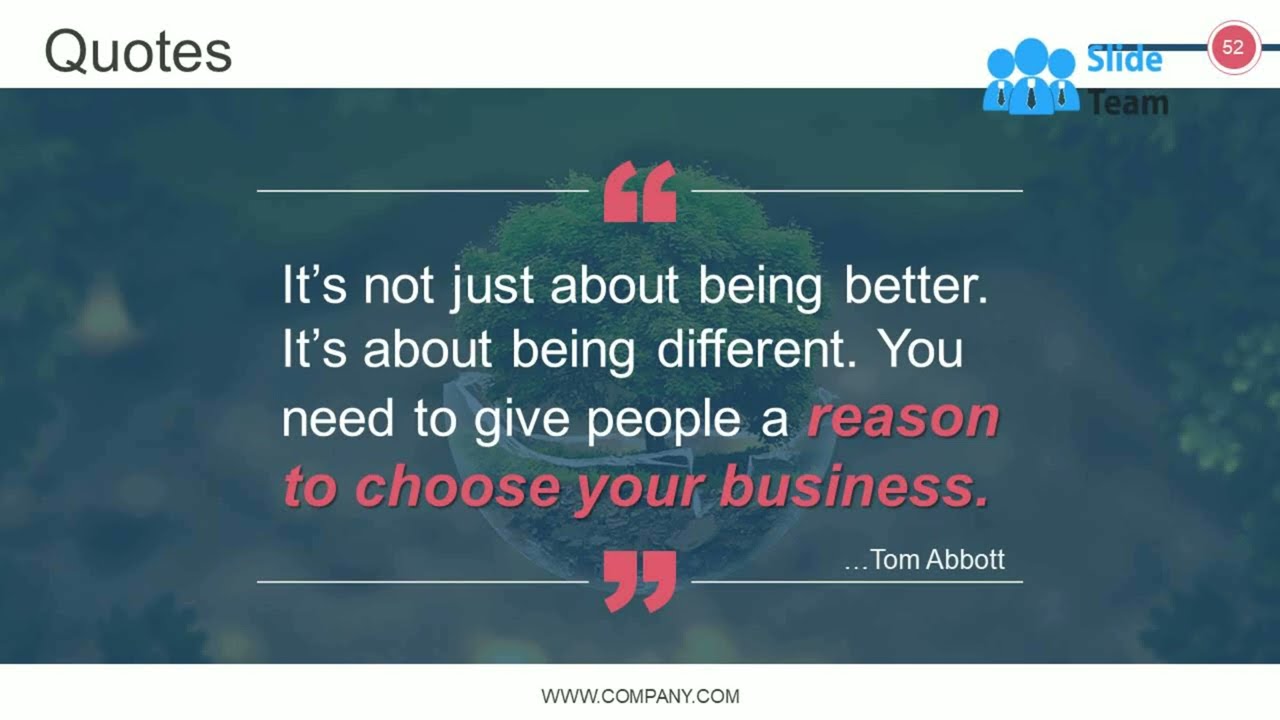The image is a slide from a larger presentation with a white bar across the top and bottom. At the top left, it reads "quotes" in black lettering, and on the right, there's a blue icon of three people wearing ties labeled "Slide Team 52." The upper right corner also features a small red circle with the number 52 inside it. The main body of the slide has a greenish-gray background with some greenery or a plant in a half-bubble vase. In the center of the slide, there's a quote highlighted in large text: "It's not just about being better, it's about being different. You need to give people a reason to choose your business." Key phrases such as "reason" and "to choose your business" are in red. The quote is attributed to Tom Abbott, with his name positioned at the bottom right of the text. Below this, along the bottom bar, there's a web address, www.company.com.